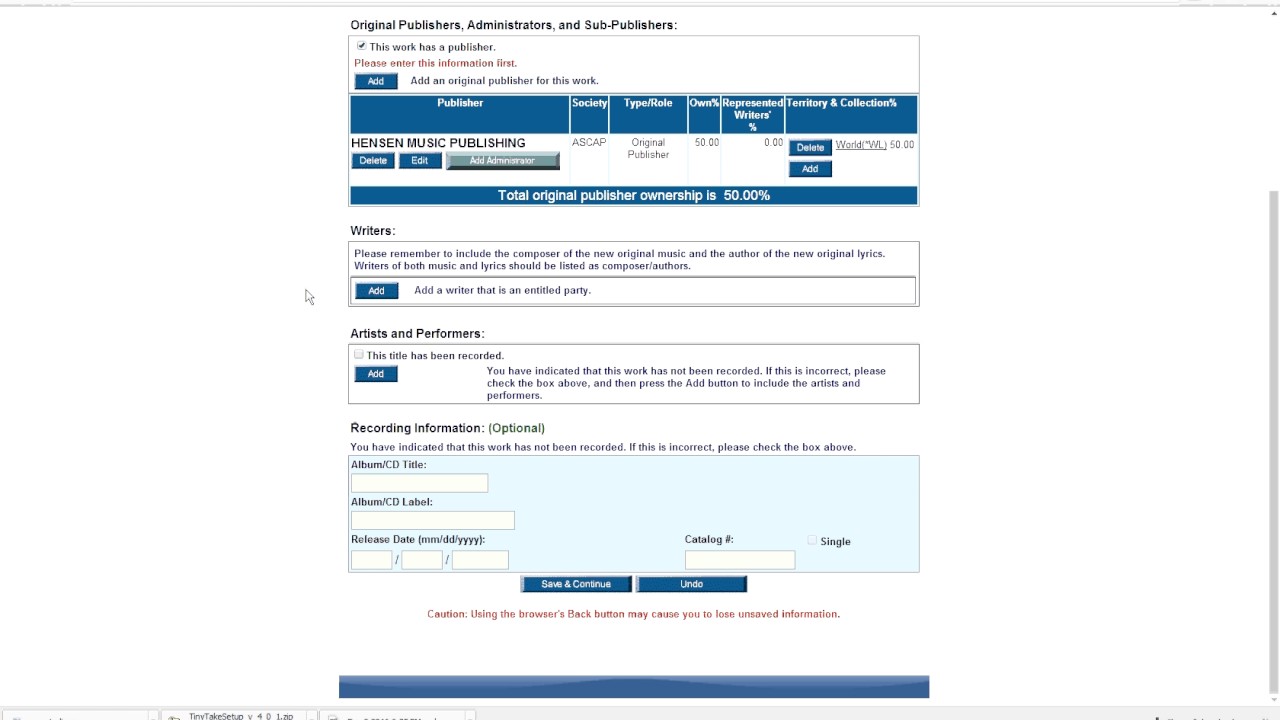The image displays a form related to publishing information, divided into various sections with a predominantly blue palette and white text, making some parts difficult to read. At the top of the image, the headers "Original Publishers," "Administrators," and "Sub-Publishers" are prominently displayed in blue. Beneath this, a box states: "This work has a publisher. Please enter this information first. Add an original publisher for this work." Inside the box, the text indicates "Publishers Henson Muser Publishing" under the section labeled "Society" with "ASCAP" specified.

Further down, there are fields requiring some type of rate entry, and the remaining columns have white letters on a blue background, making them quite challenging to decipher. Below this section, there's a note indicating that the total original publisher ownership is 50%. 

Above this, another section titled "Writers" includes text encouraging the reader to remember details about the composer of the new original series and the author of the newly originated work, although this part is particularly illegible due to its small, purple font. This section also contains a blue "Add" button, as well as a button for adding a third-party webcam, although the details here are somewhat unclear.

There is a segment labeled "Artists and Performance" which verifies that "This site has been recorded," followed by an additional line in purple that is difficult to read. Below this, another informative section in green, titled "Recording Information (optional)," allows the inclusion of additional information, all set against a blue background.

Furthermore, there are two blue boxes with white text at the bottom of the form, above a notable red statement just before the final blue bar of the image.